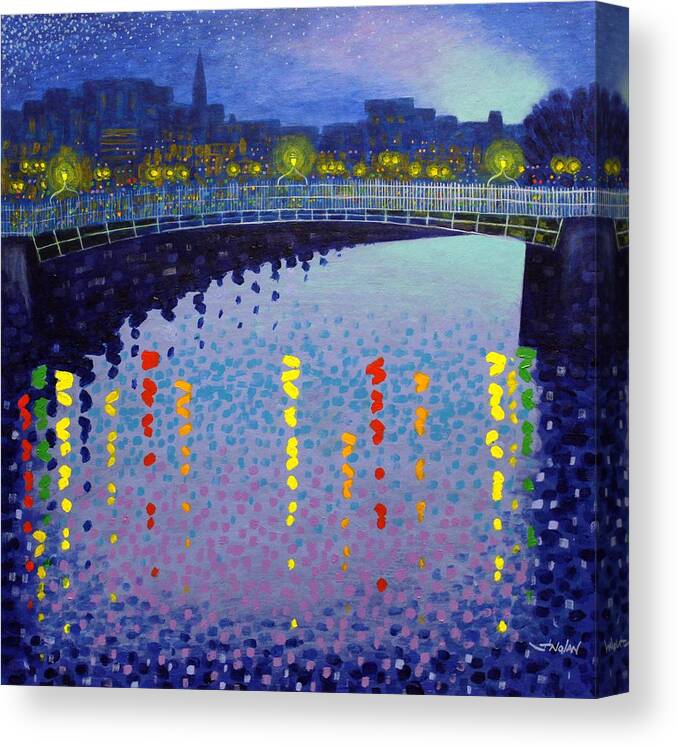This painting, executed in an impressionistic style, beautifully showcases a nighttime cityscape with a river running through it. The scene is dominated by a walking bridge adorned with bright, golden lanterns that cast a warm glow, dotting the entire span. Below, the river occupies the bottom three-quarters of the canvas and is rendered with a textured mix of light blue, dark blue, and black, with colored reflections of the bridge lights in vibrant red, orange, yellow, and green ribbons. The water also features various lighter blue and purple dots, adding to its rich, impressionistic texture. Above the bridge, a city skyline is visible with a prominent tall church tower and interspersed trees. The sky, a kaleidoscope of blue, light blue, purple, and teal hues, is studded with white stars, heightening the painting's nighttime ambiance.